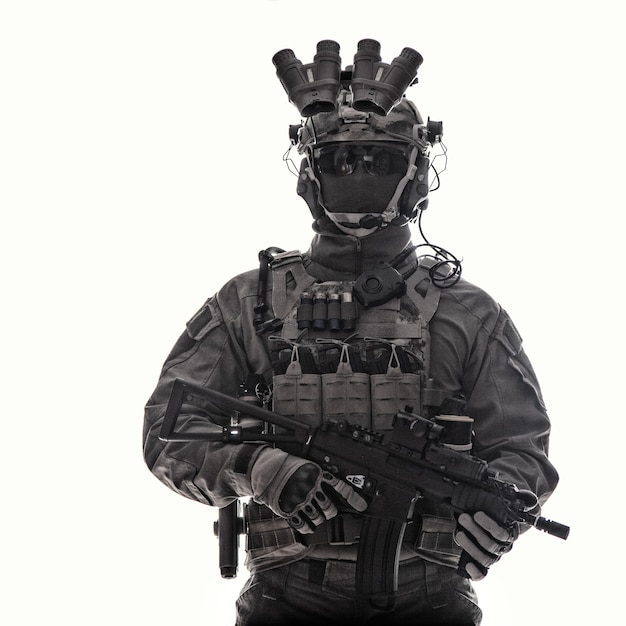This highly detailed black-and-white photograph captures a formidable soldier or high-level security operative, exuding a distinctly ominous and tactical presence. The individual, whose gender is indiscernible due to their full face covering, is decked out in advanced combat gear from head to waist. They wear a camouflage-patterned helmet featuring dual cylindrical attachments, likely night vision goggles, angled above the forehead, and a myriad of straps securing various equipment. Dark sunglasses shield their eyes while a tightly wrapped scarf completely covers their mouth, adding to the air of anonymity. 

Beneath the neck, the soldier has an array of ammunition holders, with four visible bullet holders, and a microphone positioned on the right side, suggesting extensive communication capabilities. Their puffy, heavy-duty jacket underpins a tactical vest laden with multiple pockets and essential gear. Wires snake down from their helmet past their ears, connecting to various devices. The dark, utilitarian color palette of black, gray, and tan enhances the overall foreboding aesthetic.

In their gloved hands, they firmly grip a submachine gun, described by some as similar to an AK-47, hinting at a collapsible stock and clip ready for action. The soldier's attire is completed by black tactical pants and an ammo belt, showcasing readiness and resilience. Positioned against a very light cream square background, the complete absence of environmental context draws full attention to this intimidating, well-equipped individual, poised for tactical operations.